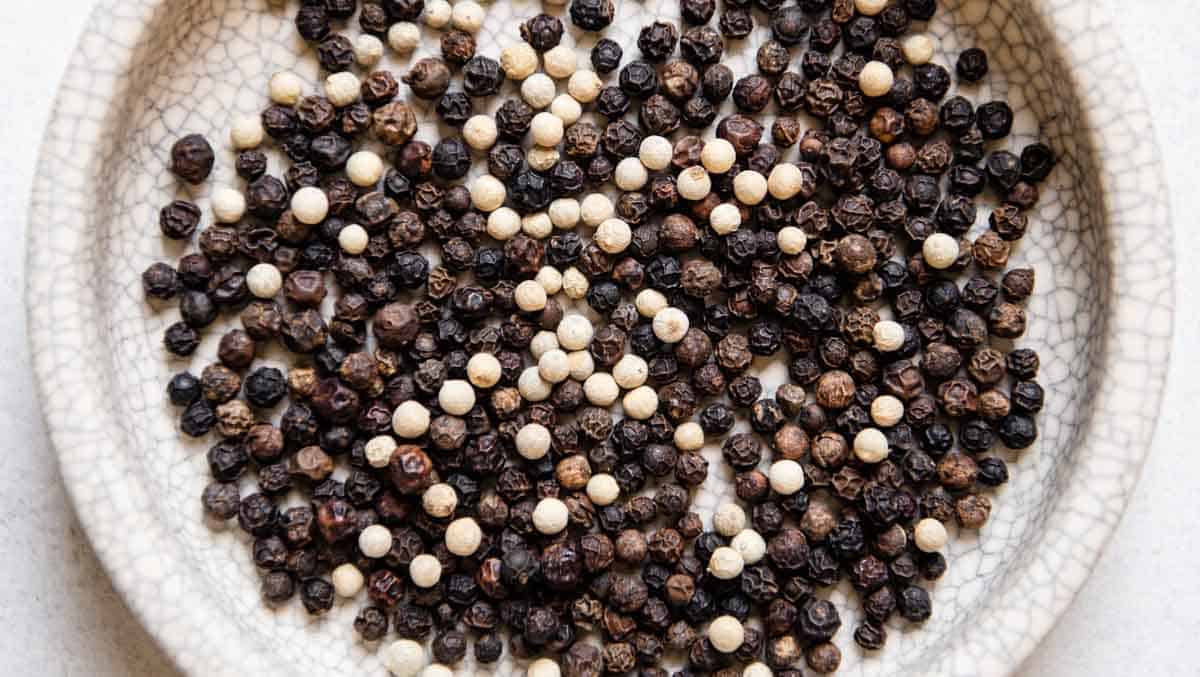The image is a detailed color photograph featuring an assortment of peppercorns in various shades and a few cloves arranged in a shallow, round, white porcelain dish. The dish is notable for its intricate crackle glaze, giving it a unique textured appearance. The peppercorns, which range in color from black, brown, and dark orange to cream and white, are randomly scattered, suggesting a natural, unarranged composition, though the white peppercorns appear predominantly on top, hinting at a possible deliberate placement for contrast. The entire arrangement sits on a white table, creating a clean, monochromatic background that emphasizes the vibrant, earthy tones of the peppercorns and cloves. Overall, the image captures a close-up view of this colorful medley, accentuating the textures and hues against the simple backdrop.